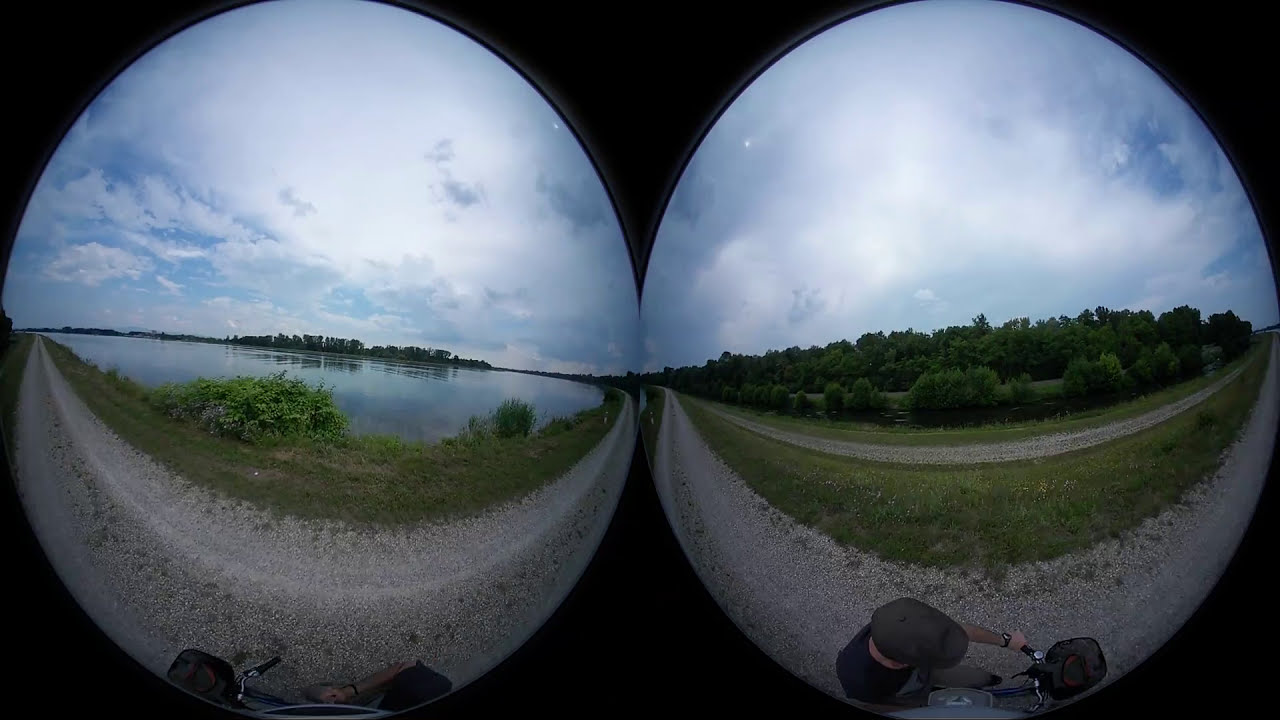The image features a 360-degree panoramic view presented as two fisheye lens "globes," offering a unique and immersive perspective. The left globe unfolds a serene lake scene; the water is a calm, smooth gray under a sky filled with gray and white clouds, allowing glimpses of blue. Along the horizon, a line of vegetation, primarily trees, stretches across the center, becoming lower towards the edges. A green shrub sits prominently at the water's edge in the foreground. A winding dirt and gravel road curves from the left, sweeps down, and then turns right, looping back to the top of the globe.

Contrastingly, the right globe displays a dense canopy of green trees under a similarly cloud-dotted sky with specks of blue on the right. A gray path meanders through the greenery, encircled by grass and looping back into the trees. The bottom of this globe features a man on a bicycle. He dons a gray flat cap, black shirt, and wristwatch, with his hands visible on the chrome handlebars, which have a black handlebar bag hanging from them. He rides along what appears to be a small, gravelly road amidst this lush scenery.

Together, these globes create a vivid and detailed depiction of a tranquil and picturesque location, rich in natural beauty and possibly a popular scenic or tourist spot.